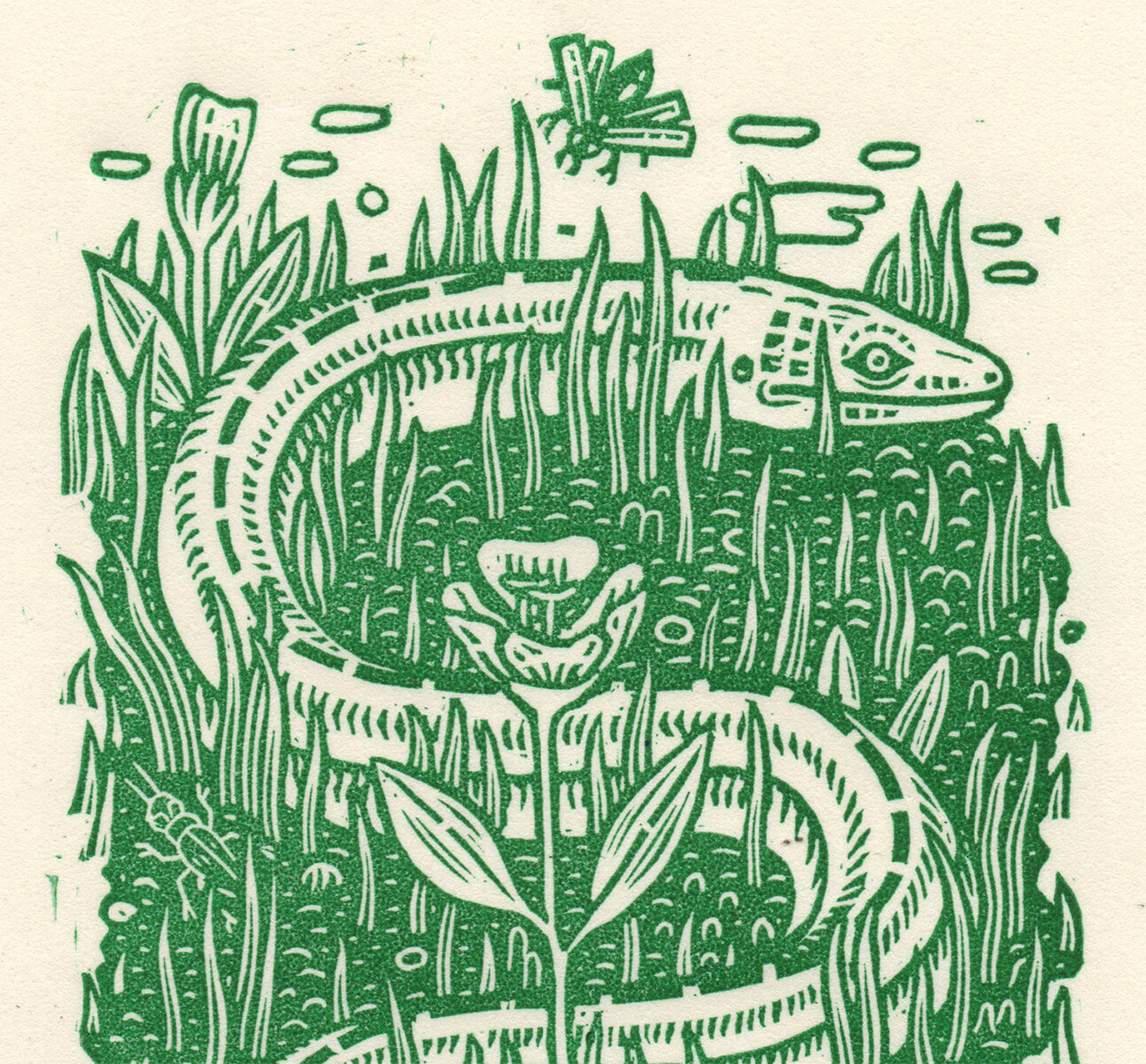The image is a monochromatic, green and white illustration of a snake coiled in an S-shape, slithering through dense grass dotted with flowers. The snake has a neutral expression with distinct green stripes and dashed lines on its white body, emphasizing its features and face. The scene has a simple, cartoonish style reminiscent of antique children's book illustrations. The lush green grass, highlighted with white outlines and interspersed with flowers, surrounds the snake. A small green fly hovers above the snake's head against a white background, adding to the whimsical and naive quality of the illustration. Moreover, there are subtle hints of water with possible lily pads in the background, completing this quaint, vintage depiction of nature.